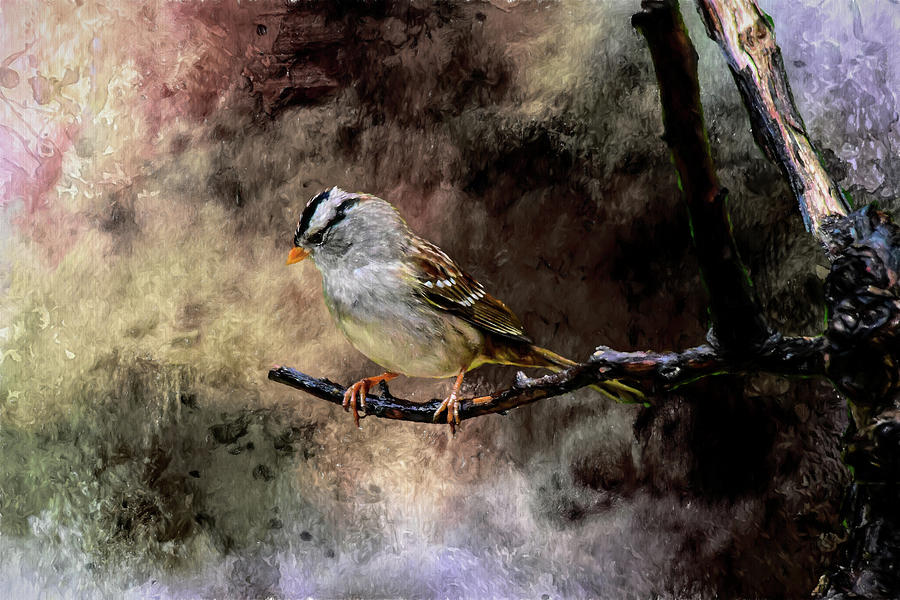This oil painting portrays a small bird, likely a finch, perched on a leafless branch, which gives the impression of having been damaged or burnt, contributing to the painting's gloomy feel. The branch extends from a tree situated on the right side of the frame. The bird, centered and stationary, is depicted in a three-quarter view, gazing downwards to its right. The finely detailed bird has a whitish breast, a distinct orange beak, and a crown featuring black and white stripes. Its brown feathers, tipped in white, extend to a narrow greenish-yellow tail. The bird's little orange feet firmly clutch the branch, adding to the intricate realism. The background is an abstract mix of blacks, purples, whites, and bluish tints, merging with occasional lighter browns, tans, and hints of darker greens, enhancing the overall somber tone of the painting and suggesting an environment affected by a calamity, like a forest fire.